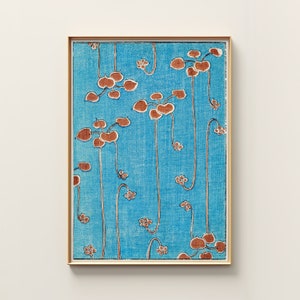The image is a small, abstract art piece with a grayish pink, very light background resembling fabric, possibly textile or embroidery. It features a narrow, light gold frame around the artwork. The scene primarily uses a robin's egg blue for the backdrop, simulating the sky. The composition includes red and white flowers with heart-shaped, cream-outlined petals. These flowers are connected by delicate white stems that resemble thin yarn. Scattered throughout the piece are tiny flower blooms, suggesting new growth. The flowers and stems are depicted in sandy, brownish hues, adding to the intricate, textured feel of the image. The overall effect is a surreal, almost whimsical depiction of flowers, with an abstract flair reflective of both sky and perhaps underwater elements.